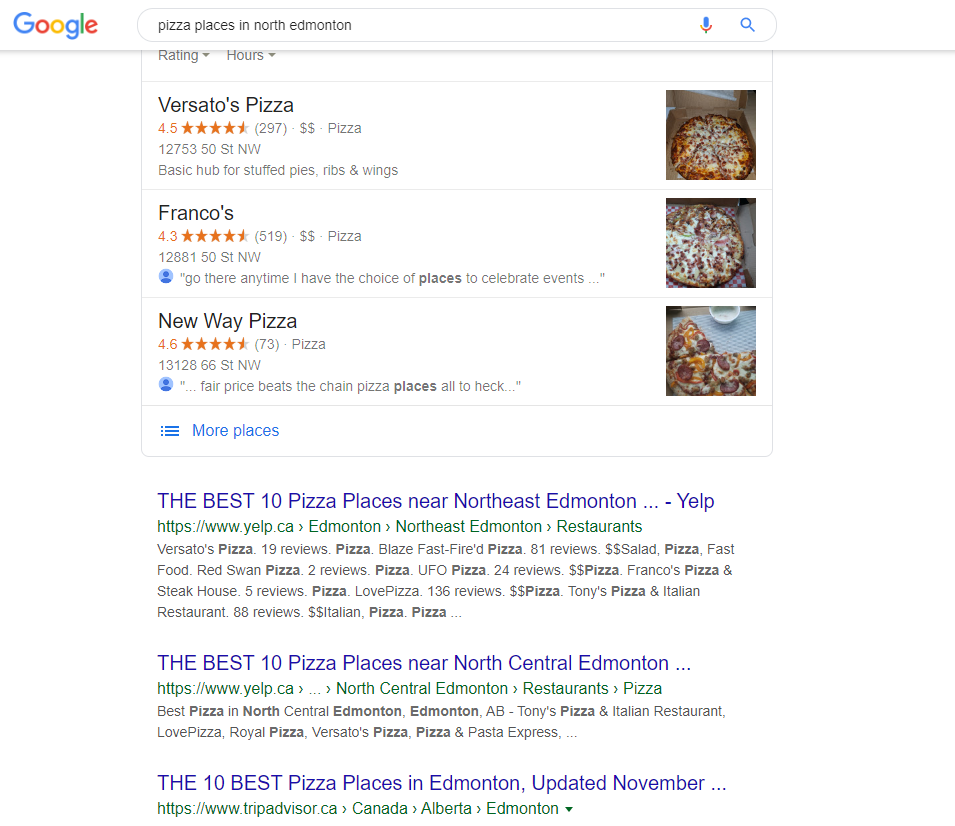This image captures a Google search results page for "pizza places in North Edmonton." In the top left corner, the familiar Google logo is visible. The search bar at the top contains the query "pizza places in North Edmonton." Below it, various search results are listed.

The first result showcases "Versado's Pizza" with a rating of 4.5 stars. It includes the address and a brief description: "Basic hub for stuffed pies, ribs, and wings." To the right, there's a mouth-watering photo of a pizza.

The second result highlights "Franco's," which boasts a 4.3-star rating. The address is provided, and a review snippet reads, "Go there anytime I have the choice of places to celebrate events." Beside this entry is another enticing photo of a pizza.

The third result features "New Way Pizza," rated at 4.6 stars. Along with the address, it includes a review stating, "Fair price beats the chain pizza places all to heck." Accompanying this listing is a photo of a partially-eaten pizza, adding to the anticipation.

Further down, another search entry reads, "The best 10 pizza places near northeast Edmonton Yelp," followed by a Yelp link and a list of various restaurants including Versado’s Pizza, Blaze Fast-Fired Pizza, and UFO Pizza.

The next result states, "The best 10 pizza places near north central Edmonton," followed by a web address and mentions "north central Edmonton restaurants pizza."

Finally, the last search result on the page appears as "The 10 best pizza places in Edmonton updated November," with only the site address provided.

This comprehensive search results page offers a detailed guide to some of the best pizza spots in North Edmonton, complete with ratings, addresses, reviews, and delicious images.